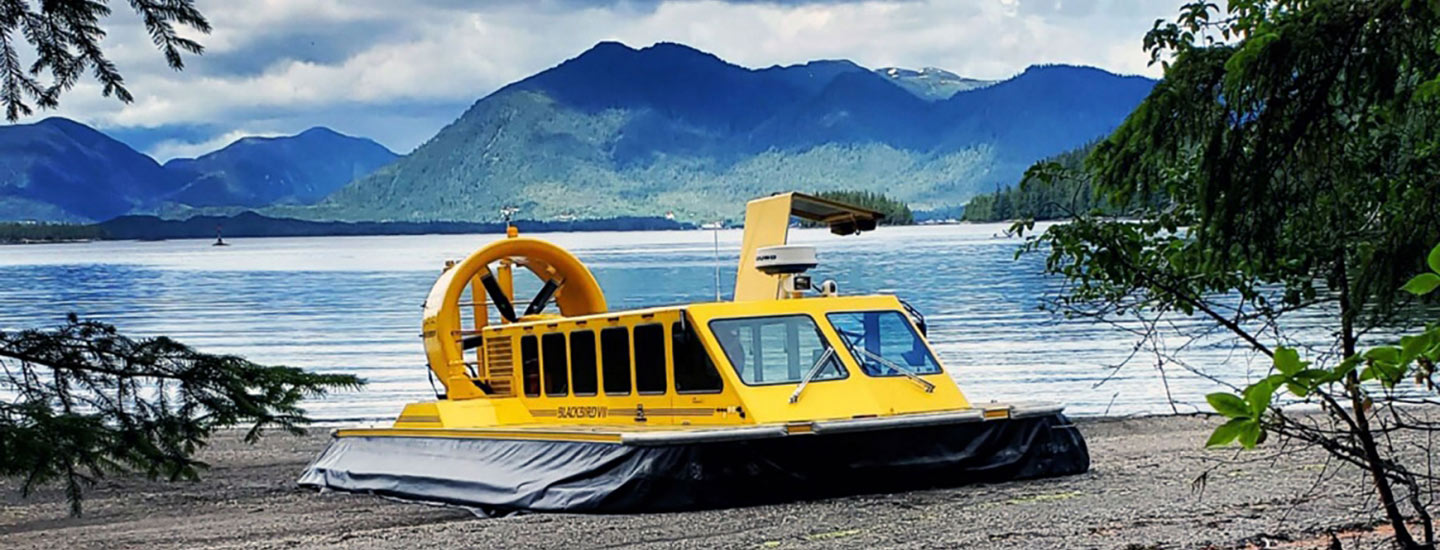The image features a bright yellow and black hovercraft, which is docked on a sandy beach. The hovercraft's rectangular body with a curved front and flat, windowed area slopes downwards toward the sand. It has large square windows on the front, and additional windows running along its sides. The bottom of the hovercraft is encased in a black tarp-like material, characteristic of its design to hover. On the back, a prominent feature is a large, circular opening housing a yellow fan blade. 

The background reveals a picturesque scene with calm blue waters and a cloudy sky, exhibiting hues of gray and white. Distant blue mountains are covered with patches of green foliage, while smaller, densely forested hill ranges filled with green pine trees frame the horizon. The beach itself has a mix of tan and gray sand, with strands of green bushes and trees flanking the hovercraft on both sides. There are no signs of people, animals, or text within the image, suggesting a still and serene atmosphere that might have been captured professionally.